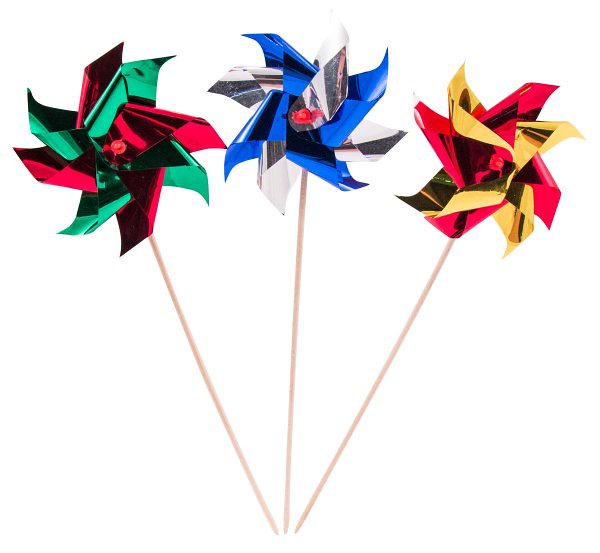The image features a set of three colorful pinwheels positioned against a stark white background. Each pinwheel is composed of shiny, reflective materials reminiscent of wrapping paper, adding an eye-catching sparkle. All three pinwheels are mounted on beige sticks, which converge at the bottom, creating a visual arrangement that resembles the shape of a 'W'. The pinwheel to the left is made of green and red materials, the one in the middle showcases a blue and silver palette with a small red pin at the center, and the pinwheel on the right is crafted from gold and red materials, also featuring a red pin at its center. The sticks on the outer pinwheels are slanted, while the middle pinwheel's stick is positioned straight, forming a triangular configuration.